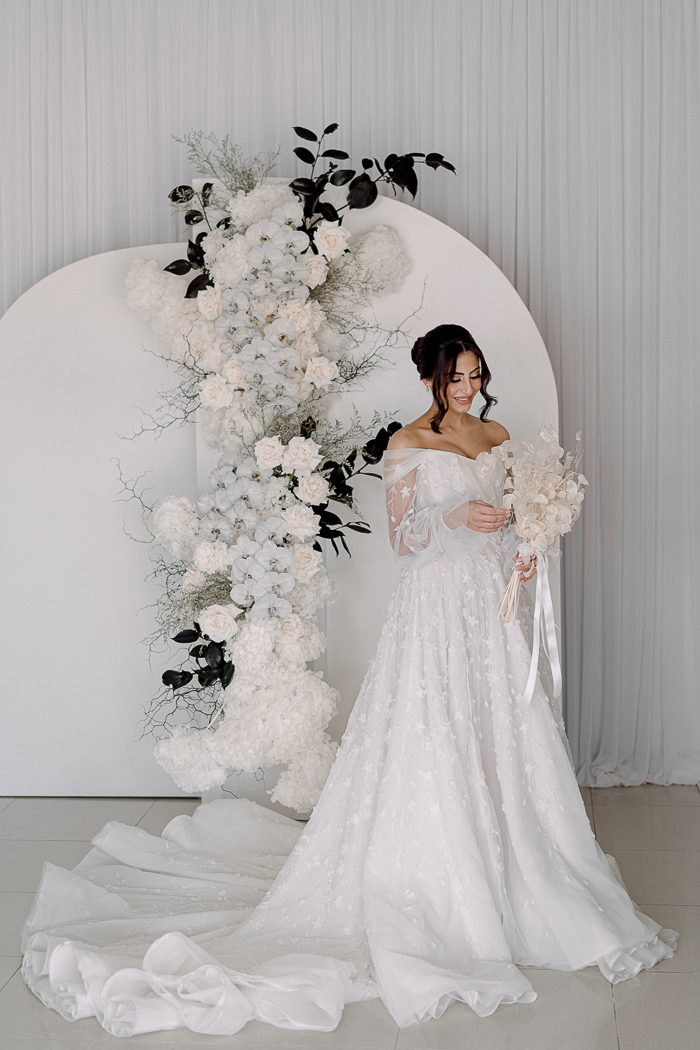A stunning bride stands gracefully on a pristine, hard surface floor, which appears to be made of concrete or tile. She is adorned in a breathtaking bridal gown that features an off-the-shoulder design with sheer lace sleeves and a slightly curved sweetheart neckline that delicately exposes the top of her breasts and neckline. The bodice is loose-fitting and flows elegantly down to the floor, extending into a moderate train that trails about three feet behind her, concealing her shoes.

Her brunette hair is styled in a chic chiffon bun, with loose tendrils softly framing her face. She gazes down with a tender smile, revealing her teeth, as she holds a bouquet of cream-colored flowers with a white ribbon elegantly draped from her hands.

Behind her, a large, white, heart-shaped structure stands against a white fabric curtain backdrop. This structure is adorned with a vertical row of white flowers interspersed with black flowers and stems, creating a striking contrast. The setting is predominantly white, exuding a sense of elegance and purity, perfect for the occasion, which could either be a wedding or a bridal shower celebration.